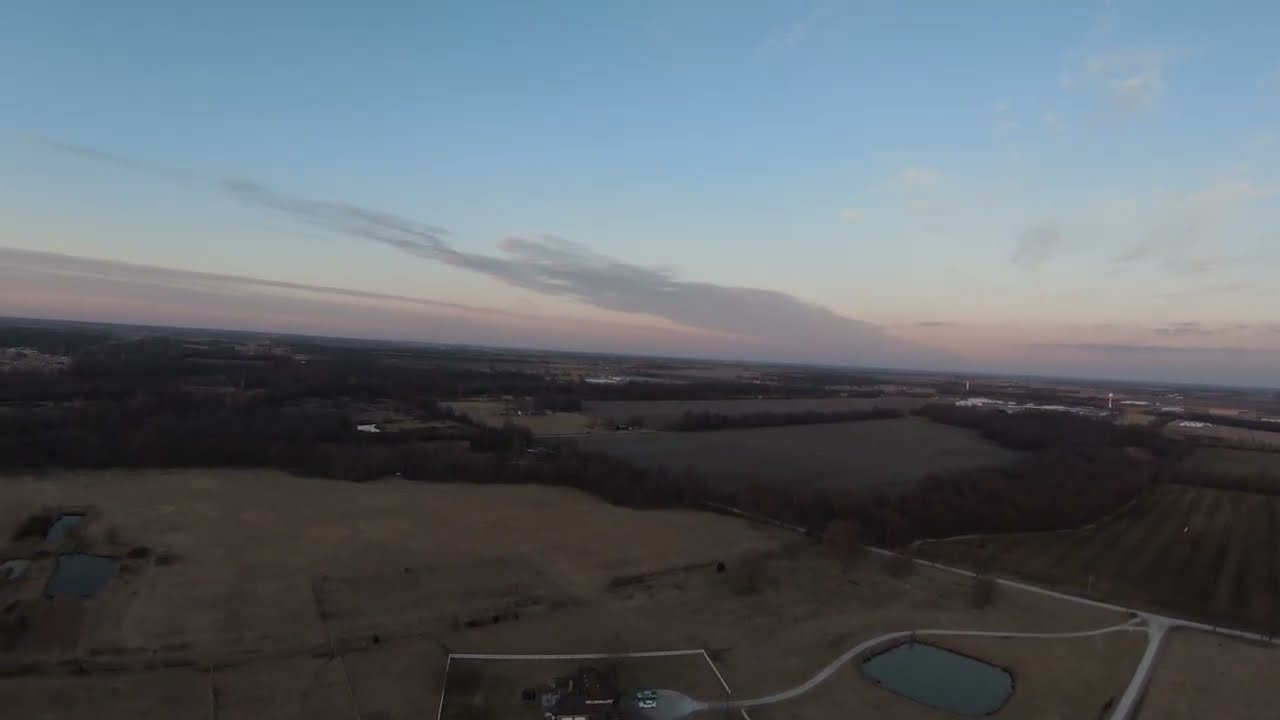The image depicts an overhead, possibly aerial, view of a sprawling landscape at dusk, with an overcast or dimly lit evening sky. The upper portion of the image reveals a mix of blue and gray hues, indicating the darkening sky. Below, the land is dominated by fields of light brown grass, interspersed with trees and bushes. Centered in the landscape is a distinctive rectangular pond with curved corners, partially framed by trees. There's also a white road, visible from above, forming an upside-down "V" shape. Most of the middle ground features large patches of dirt, adding to the varied texture of the terrain. The overall scene, though dark, conveys a vast, serene agricultural area, detailed with natural and human-made elements.